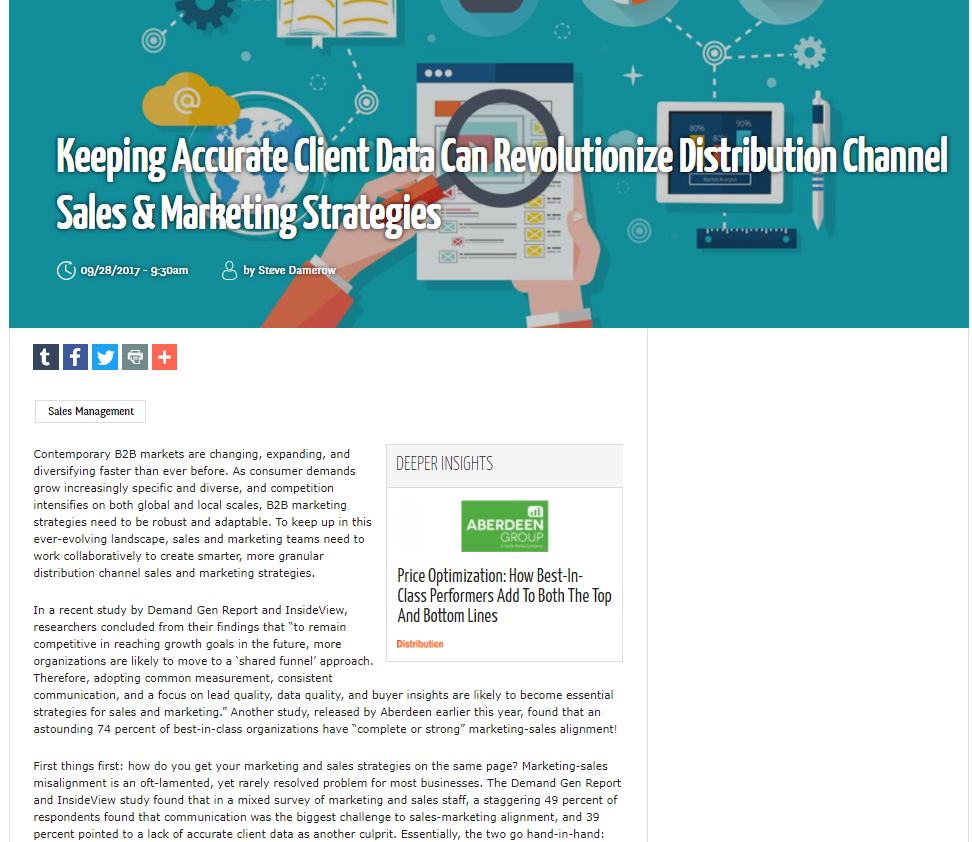The image depicts a webpage, likely a homepage, with a teal banner. The banner features images of various objects including books, wheels, a tablet, a pen, and a ruler. Additionally, there is a person depicted holding a magnifying glass in their left hand, examining a piece of paper held in their right hand. Alongside these visuals, there is an icon of a globe within a circle and a cloud symbol featuring an '@' symbol.

The main text on the banner reads in white font: "Keeping accurate client data can revolutionize distribution, channel sales, and marketing strategies." Below this text, there is a smaller segment that appears to serve as a timestamp or publication information. It reads "OG 04/09 04/28 04/20 2017 9:30 AM by Steve Damro."

The page also includes social media tabs for Tumblr, Facebook, Twitter, Google Plus, and an option to print the page. The title of the article presented on the page is "Sales Management."

On the right side of the homepage, there is an advertisement box labeled "Deeper Insights" by Aberdeen Group. The text within this advertisement promotes price optimization, stating: "How best-in-class performers add to both the top and bottom lines."